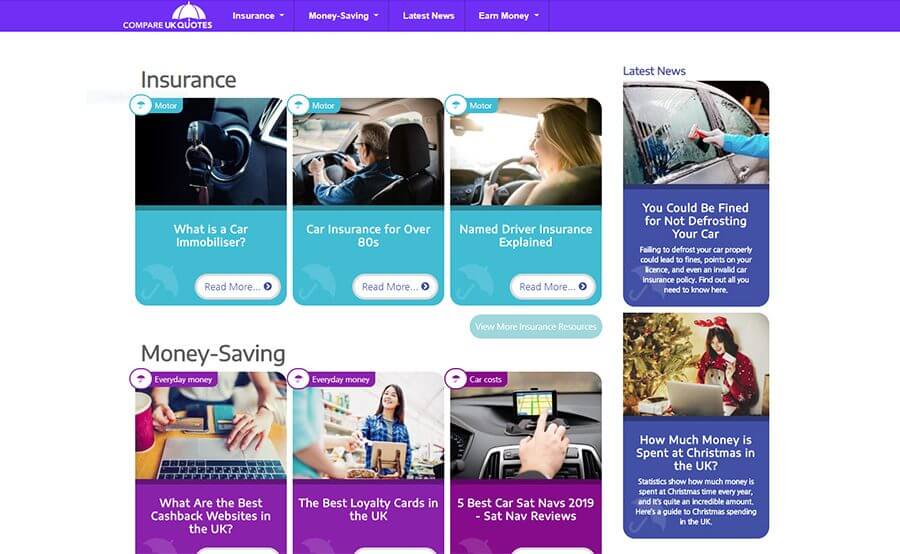This image, taken from the "Compare UK Quotes" website, features a distinct purple rectangular header with drop-down menus labeled "Insurance," "Money Saving," "Latest News," and "Earn Money." At the top center, an icon of an umbrella prominently signifies the website's logo. The background is predominantly white, creating a clean and organized layout. 

Under the "Insurance" section, three teal rectangles display images and titles: 
1. "Car Insurance for Over 80s" with a photograph of a man's hand on a steering wheel.
2. "Named Driver Insurance Explained" illustrated with a woman driving.
3. "What is a Car Immobilizer?" accompanied by an image of car keys in an ignition.

The "Money Savings" section is structured similarly with three teal rectangles:
1. "What are the Best Cashback Websites in the UK?" featuring someone looking at a computer screen.
2. "The Best Loyalty Cards in the UK" shown with a person shopping.
3. "Five Best Car Sat Navs 2019" depicted with a hand touching a smartphone on a car dashboard.

The "Latest News" section is located on the right side, maintaining a consistent design theme with taller, more vertical rectangles. Each section provides concise and relevant information, making it user-friendly and easy to navigate.